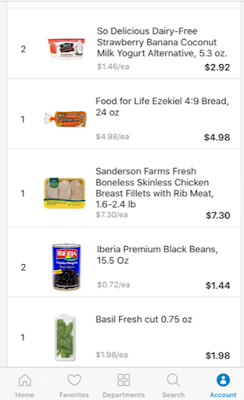Detailed caption for the shopping image:

"A screenshot of an online grocery shopping cart, featuring a variety of food items with prices and details. The list begins with two cups of a delicious dairy-free strawberry banana coconut milk yogurt alternative, each cup weighing 5.3 ounces and priced at $1.46, totaling $2.92. Next, there's a single loaf of Food for Life Ezekiel 4:9 bread, weighing 24 ounces, priced at $4.98. The cart also includes one pack of Sanders Farms fresh boneless chicken breast fillets with rib meat, with a weight range of 1.6 to 2.4 pounds, priced at $7.30. Additionally, there are two cans of Iberia premium black beans, each 15.5 ounces, priced at $0.72 each, bringing the total for the beans to $1.44. Furthermore, one package of fresh basil cut, weighing 0.75 ounces, is priced at $1.98.

The screenshot also shows functional tabs at the top for Home, Favorites, Department, Search, and Account, highlighted in blue. There are no visible indicators confirming whether this shopping is being conducted on a cell phone, tablet, computer, or through a specific grocery store or delivery service platform."